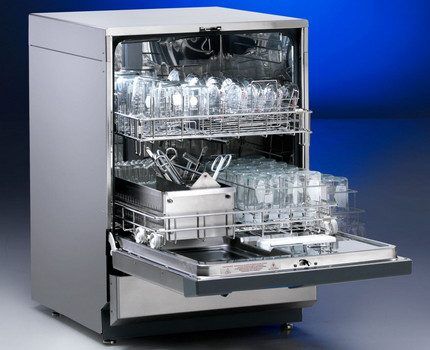The detailed image captures an open stainless steel dishwasher, prominently centered against a varying blue gradient background. The dishwasher's door is open, revealing two slightly extended trays packed with kitchen items. The top and bottom racks are loaded with glassware neatly arranged in their respective compartments. The bottom rack also contains a silverware carrier situated on the left side, holding utensils like tongs and scissors. The dishwasher stands on small legs, presenting a sturdy and realistic metallic appearance that contrasts with the deepening shades of blue in the empty background. The overall scene is portrayed with a high level of realism, emphasizing the organization and functionality of the dishwasher.